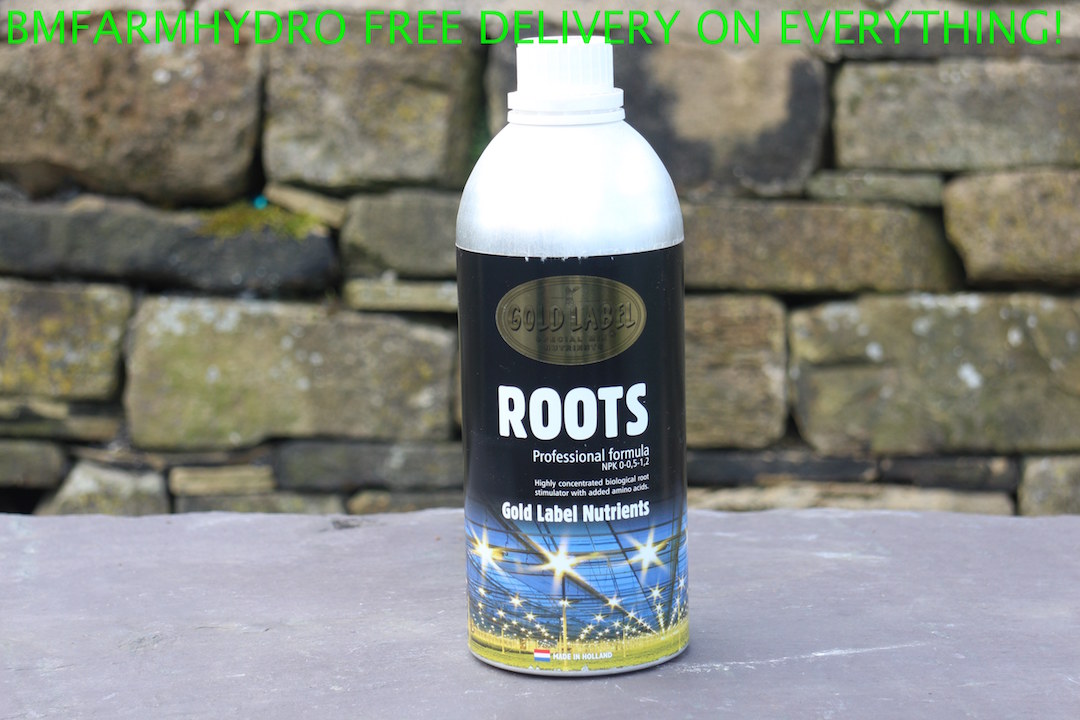This promotional photograph features a white cylindrical bottle with a white twist-off cap, prominently displayed against a dark gray and light gray stone wall. The bottle showcases a detailed label: the top half of the label has a black background, transitioning gradually to blue at the bottom. At the top of the label, there's a silver or gray horizontal oval with indiscernible text. Below this, in bold white capital letters, the word “ROOTS” is displayed, followed by a right-justified line reading “Professional Formula.” Further down, smaller white text continues, though largely unreadable, with a notable line proclaiming "Highly Concentrated Biological Root Simulator with Added Amino Acids." Near the color transition from black to blue, more bold white text reads "Gold Label Nutrients," with possible illustrations of stars or root-like imagery on the blue. The bottle rests on a flat, white or light gray surface, likely a patio table or cement path, and above it, in bright green all-caps lettering, the text “BM Farm Hydro Free Delivery on everything!” spans the width of the image.